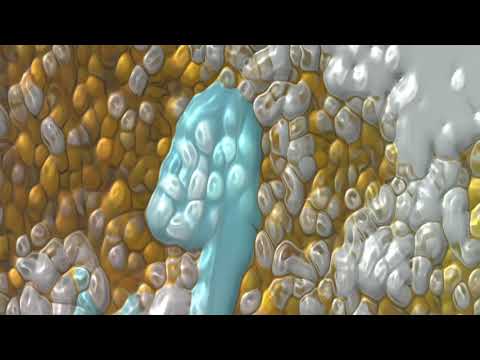The image features an abstract, possibly computer-generated depiction that resembles a microscopic view of cells or a chemical substance. Predominantly showcasing hues of yellow, white, and blue, the composition is filled with shiny, almost liquid-like blobs. The center of the image is dominated by a blue shape, which strikingly resembles an abstract horse's head or the number 4, surrounded by smaller white cellular structures. The bulk of the right side is overtaken by a large white, shiny substance, while yellow, kernel-or corn-shaped cells populate most of the left side. Despite its detailed and vivid portrayal, the exact nature of the image—whether it represents biological cells, an artistic tile or stone artwork, or a digital creation—remains ambiguous.